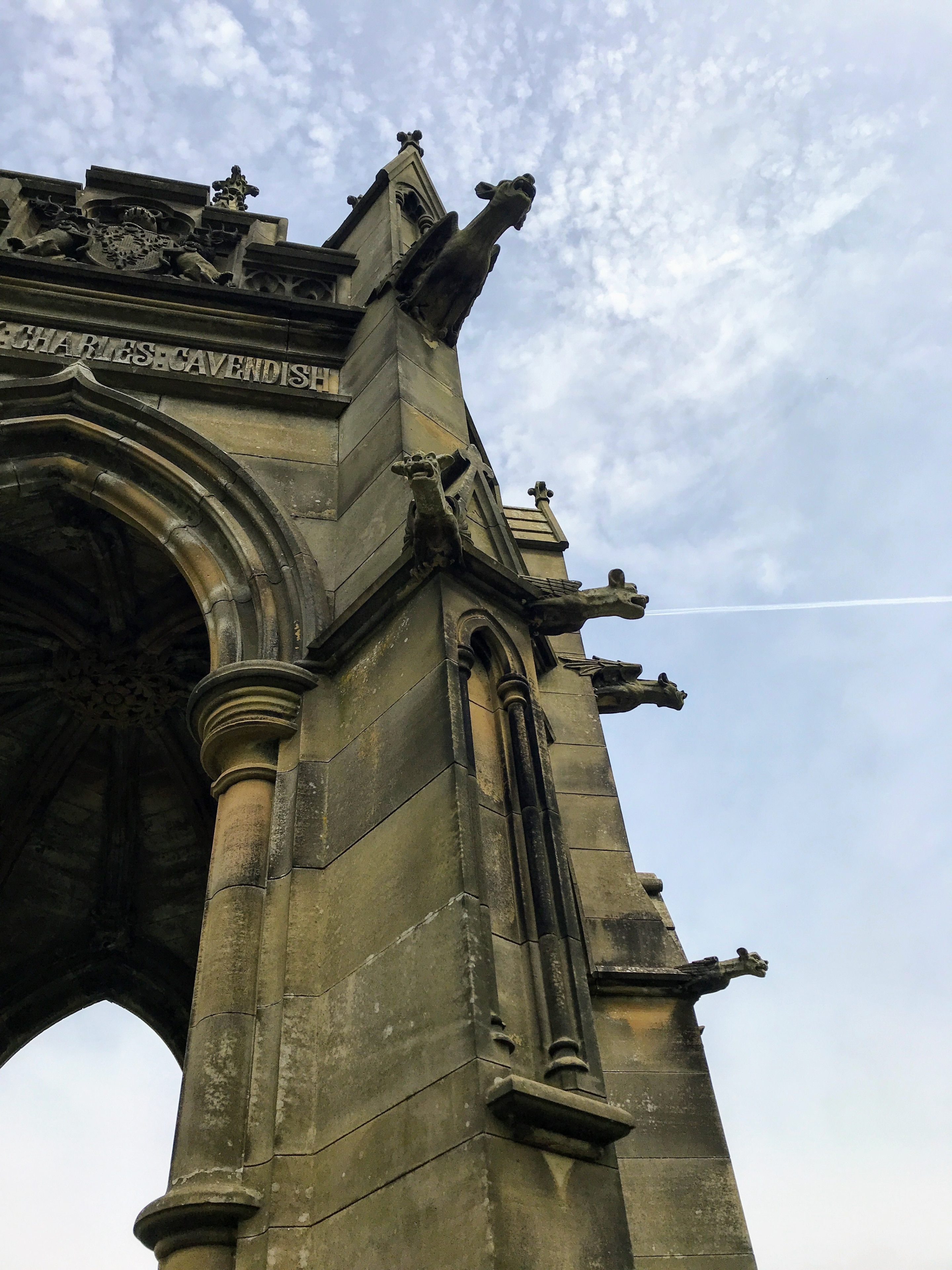The image depicts the side view of a grand cathedral in France under a clear, partly blue and white sky. The architectural structure resembles an expansive stone gazebo or tower, with intricate details including a prominent arch at its center. Above the arch, a horizontal bar bears the inscription "Charles Cavendish," with additional text partially cut off from the frame. Atop this inscription sits a statue of a person in a relaxed, seated posture, legs spread apart. Surrounding the monument are several decorative gargoyles; one is perched just above the top right corner of the arch, while two more are positioned below it on the right. The sky in the background features a distinct plane trail cutting through the clouds.